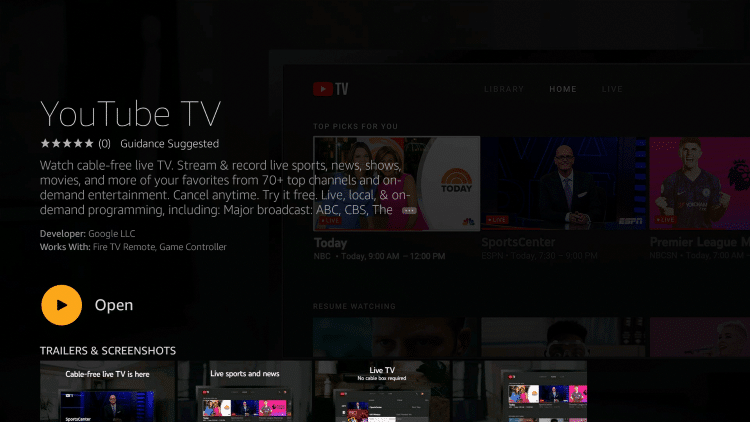This screenshot captures a web page detailing YouTube TV, presented against a predominantly black background. Behind the foreground elements, you can discern blurred thumbnails which subtly hint at the platform's diverse offerings. At the top, bold text proudly displays "YouTube TV," accompanied by a striking five-star rating and the advisory text "guidance suggested."

The promotional copy reads: "Watch cable-free live TV. Stream and record live sports, news shows, movies, and more of your favorites from 70 plus top channels and on-demand entertainment." It also highlights the service's flexibility with the phrases "Cancel any time" and "Try it free."

The page further describes the varied content available, including "live, local, and on-demand programming," featuring major broadcast channels such as ABC, CBS, and more, indicated by the partially obscured text "V dot dot dot." The developer of the service is identified as Google LLC, and a note specifies its compatibility with Fire TV remotes and game controllers.

At the bottom of the page, a row of four partly visible screenshots provides a glimpse into the user interface and visual experience, each cut off halfway down, adding a layered and engaging visual effect to the web page overview.